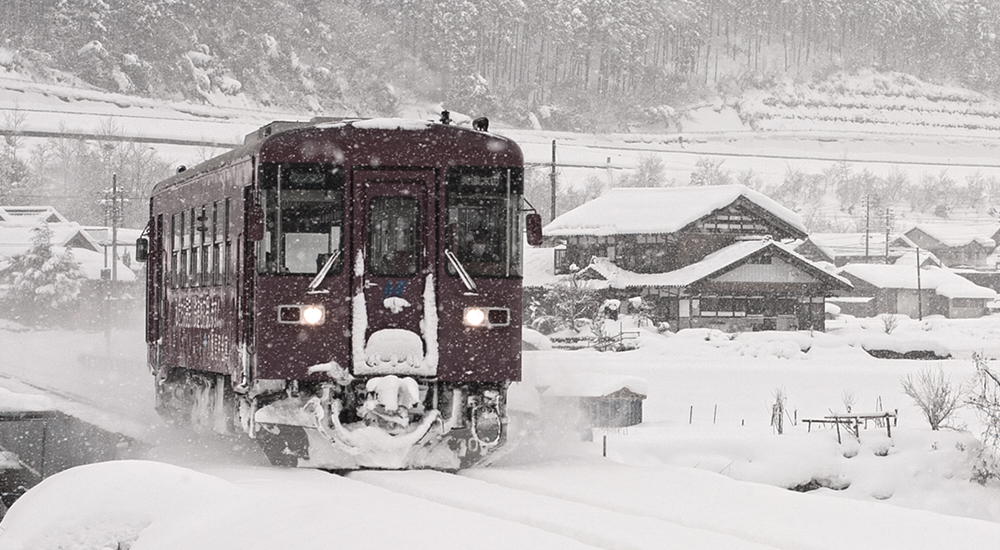This photograph captures a maroon-colored tram car gliding through a thick snowfall on snow-covered tracks. The tram, slightly left of center in the composition, appears to be coming toward the viewer, heading towards the lower right of the image. Its headlights are on, and snow billows from the tracks, emphasizing its forward motion. The vehicle features large windows along its side, with a central door flanked by smaller windows at the front. White writing is faintly visible along its side, though unreadable. 

Surrounding the tram, the snow blankets the entire scene. In the distance, there's a dense forest with a hillside draped in snow, ascending vertically to the top edge of the image. Buildings and houses with snow-laden roofs dot the background, with power lines and light poles cutting through the scene. On the right, you can see a more distinct downward hill and what appears to be a fence extending from a distant building. To the left, near the bottom corner, there's something resembling a truck bed almost engulfed by the white landscape. The photograph is dotted with thick, heavy snowflakes, reinforcing the serene yet intense winter atmosphere.